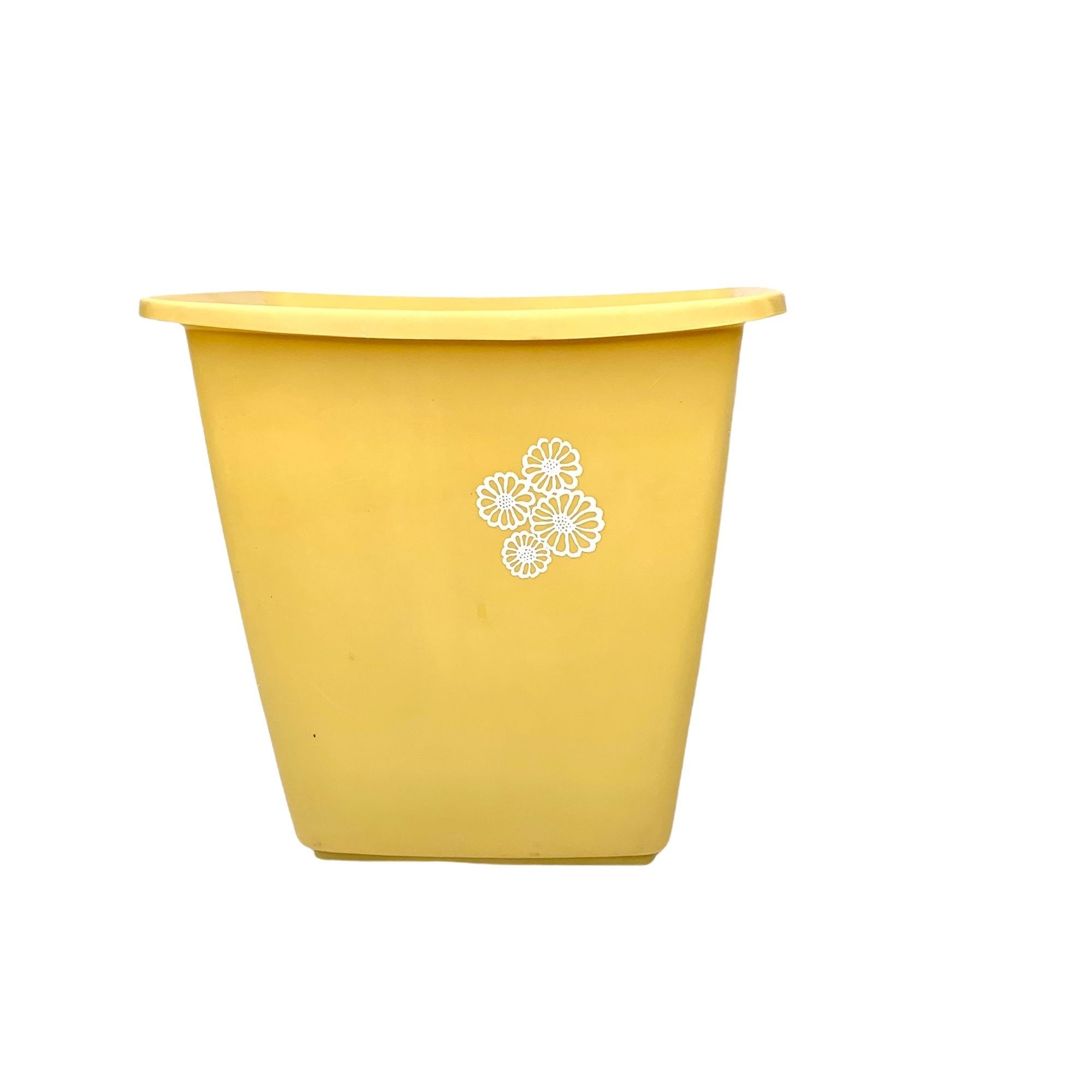This product photo showcases a minimalistic yellow trash can set against a clean white background. The image is evenly and softly lit, creating a refined and uncluttered aesthetic. The can features delicate white outline illustrations of four flowers in varying sizes, positioned in the top right corner. Its design is distinctive, with a slightly curved upper section and a trapezoidal shape that tapers towards a smaller base. The wide opening contrasts the narrower bottom, enhancing its modern look. Subtle shadows on the ground suggest overhead lighting, adding depth and dimension to the photograph.